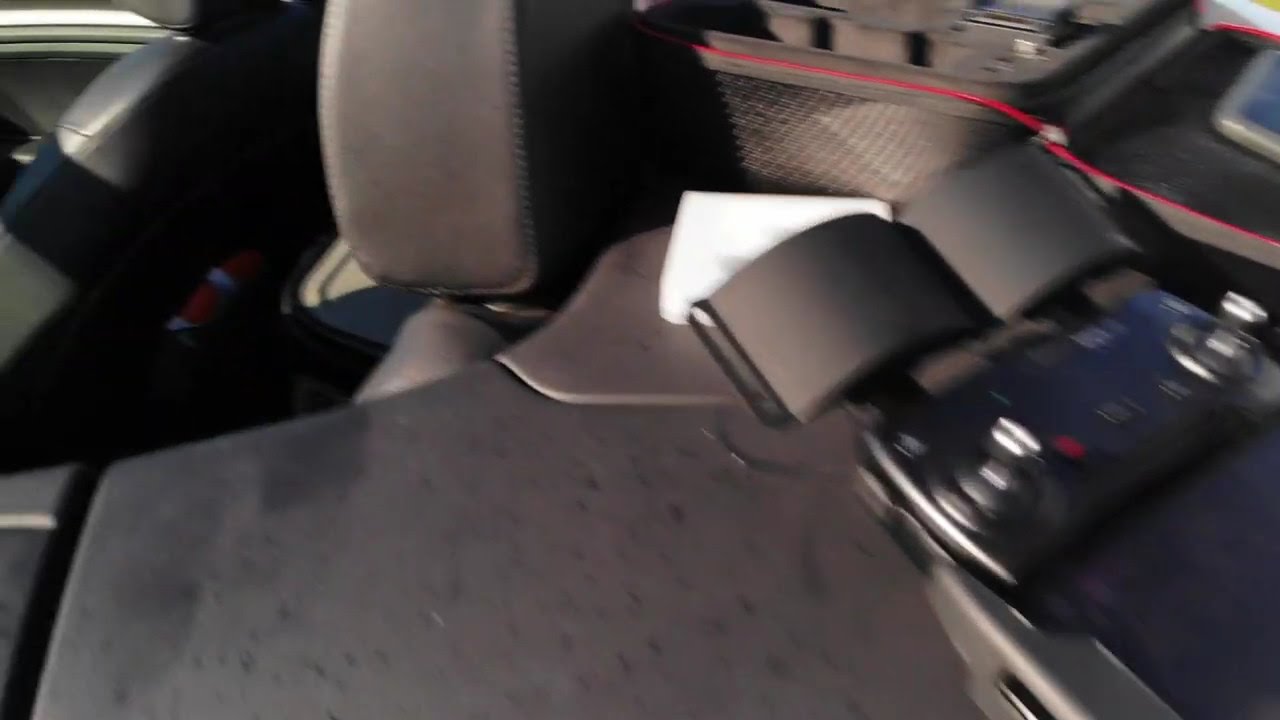The image is a close-up shot, predominantly blurry and difficult to interpret. It appears to be taken from inside a vehicle, potentially focusing on the rear or passenger seat area. The color palette is primarily brown and black, adding to the indistinct atmosphere. A cargo net seems to stretch across the middle, possibly accompanied by armrests or handrests within the car's interior. In the foreground, there is a black, square-shaped object on the lower right, likely a video game controller with two silver knobs and a red button. Another notable element is a red line that runs through the image, and there might be a speaker or remote in the background. The overall dimness and blurriness make it challenging to discern the specific details and objects clearly.